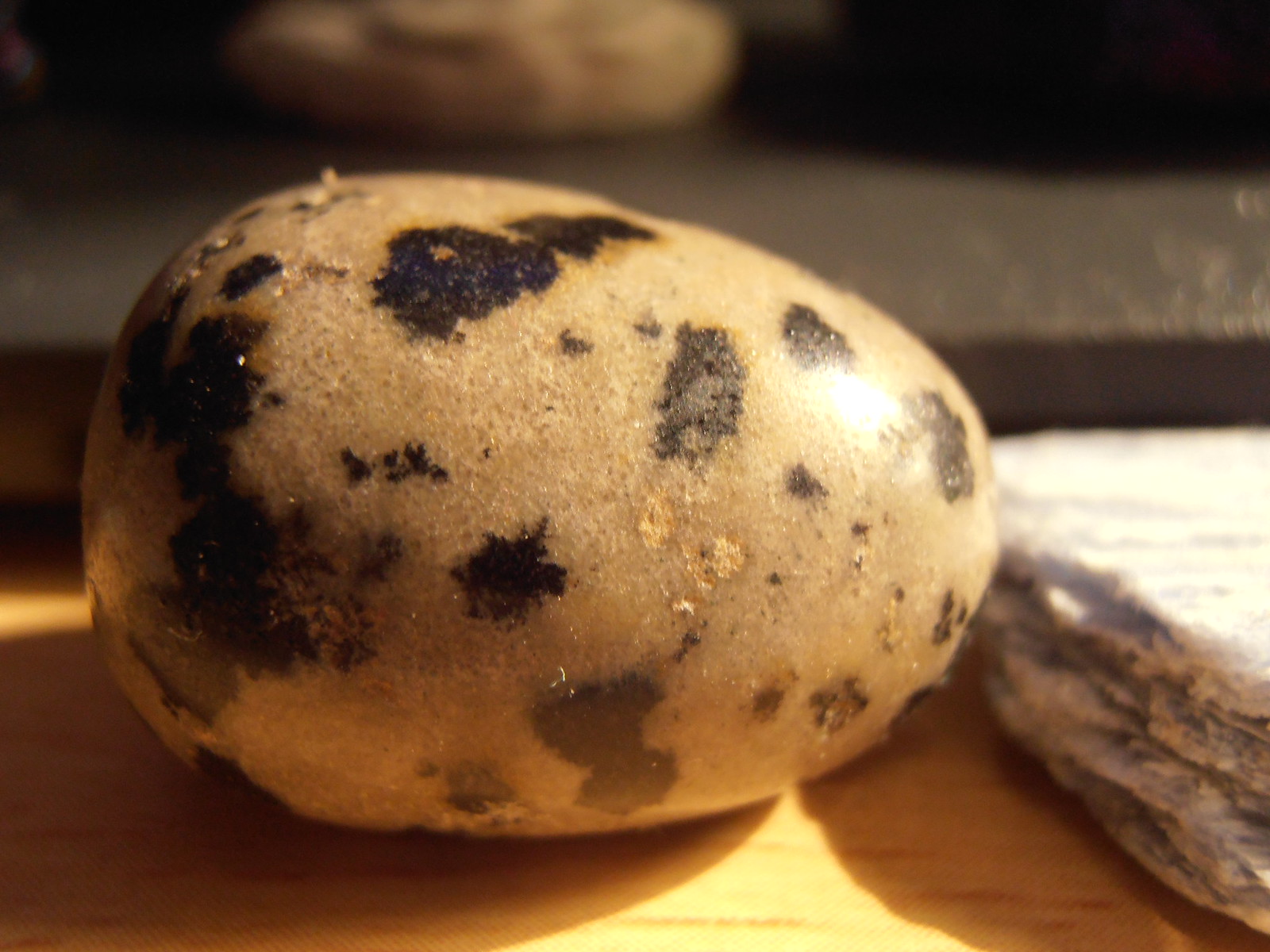The image showcases a close-up, detailed view of a spotted, round object, likely a potato or a speckled egg, lying on its side on a light wooden plank. The object, predominantly light beige with dark brown splotches, is positioned next to a large rock. The speckles are more concentrated on the left side, suggesting an uneven distribution. There are noticeable chips on the surface. Reflected in the background, possibly in a mirror, is a blurred shadowy gray scene, enhancing the worn and rugged texture of the subject. Shadows cast underneath add depth to the composition.